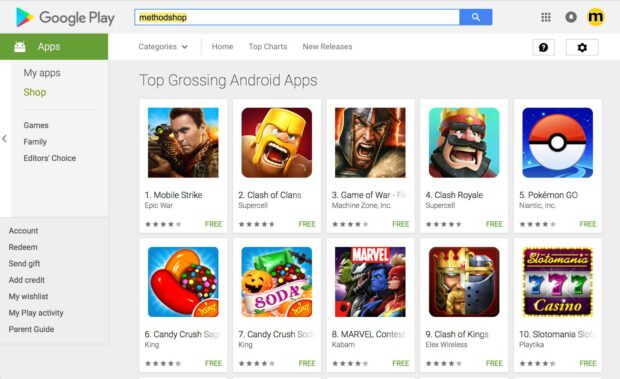A screenshot of the Google Play Store interface captures the familiar layout, featuring the following distinctive elements:

At the very top, the Google Play icon is prominently displayed beside the text "Google Play." Directly below this, a search bar contains the term "method shop" within it, accompanied by a white magnifying glass and a blue button on the right. Adjacent to the search bar, there is an icon consisting of three vertical dots arranged in three columns and three rows.

Further down, on the left side of the screen, a comprehensive menu is visible, listing numerous options: Apps, My Apps, Shop, Games, Family, Editor's Choice, Account, Redeem, Send Gift, Add Credit, My Wishlist, My Play Activity, and Parent Guide. On the right side of the screen, the top section encompasses a menu with a categories dropdown, alongside tabs for Home, Top Charts, and New Releases. At the far right of this section are two additional icons: a cloud icon possibly containing a question mark and a gear icon.

Beneath this, the top row is dedicated to Android apps, organized in a grid format of five columns and two rows, showcasing a selection of popular applications. The image overall is slightly pixelated, making some finer details less discernible, but key elements like the menus, icons, and layout are clearly recognizable.